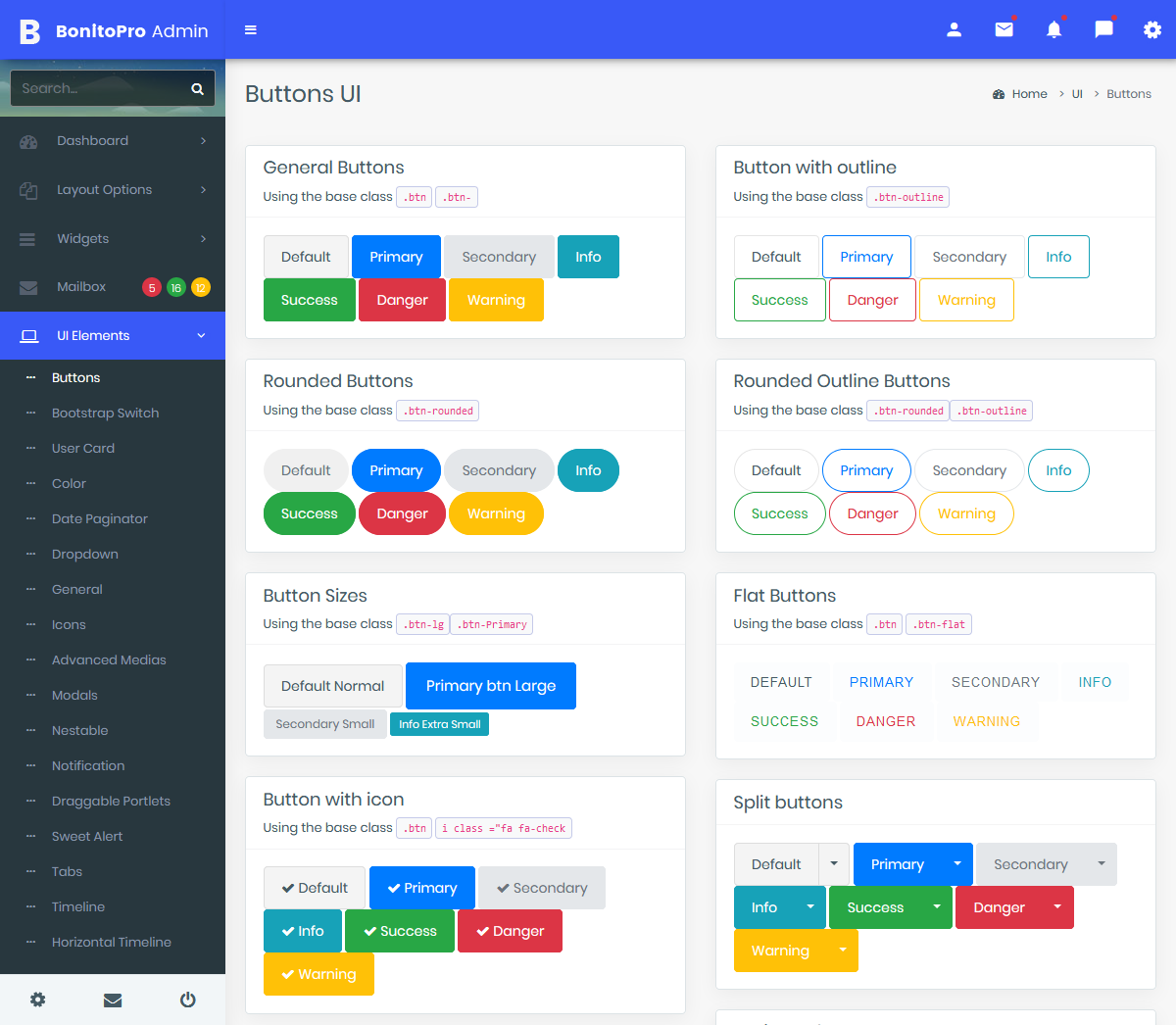The image showcases a comprehensive snapshot of the "Bon ITO Pro Admin" dashboard. Dominating the left-hand side, a large, bold, and white "B" rendered in an almost word art style stands out. Below the "B," a vertical pane forms the main navigation menu, starting with a search bar denoted by a white search icon on a mossy light green background. The remainder of the pane is predominantly black, listing several menu items including Dashboard, Layout Options, Widgets, and Mailbox. Unique indicators highlight Mailbox with three numbers: 5 in red, 18 in green, and 12 in bright yellow, reflecting a colorful categorization evident on the right side of the screen.

Further down the navigation pane, the UI Elements section is expanded, displaying a detailed list of features such as Buttons, Bootstrap Switch, User Card, Color, Date, Paginator, Drop-down, General Icons, Advanced Medias, Modals, Nest Table, Notification, Draggable, Portlets, SweetAlert, Tabs, Timeline, and Horizontal Timeline.

On the right-hand side, a detailed area presents various button configurations under multiple categories including General Buttons, Button with Outline, Rounded Buttons, Rounded Outline Buttons, Button Sizes, Flat Buttons, Button with Icons, and Split Buttons. Each button type is represented in different styles marked as Default, Primary, Secondary, Info, Success, Danger, and Warning, either partially colored, uncolored, or outlined in their respective hues.